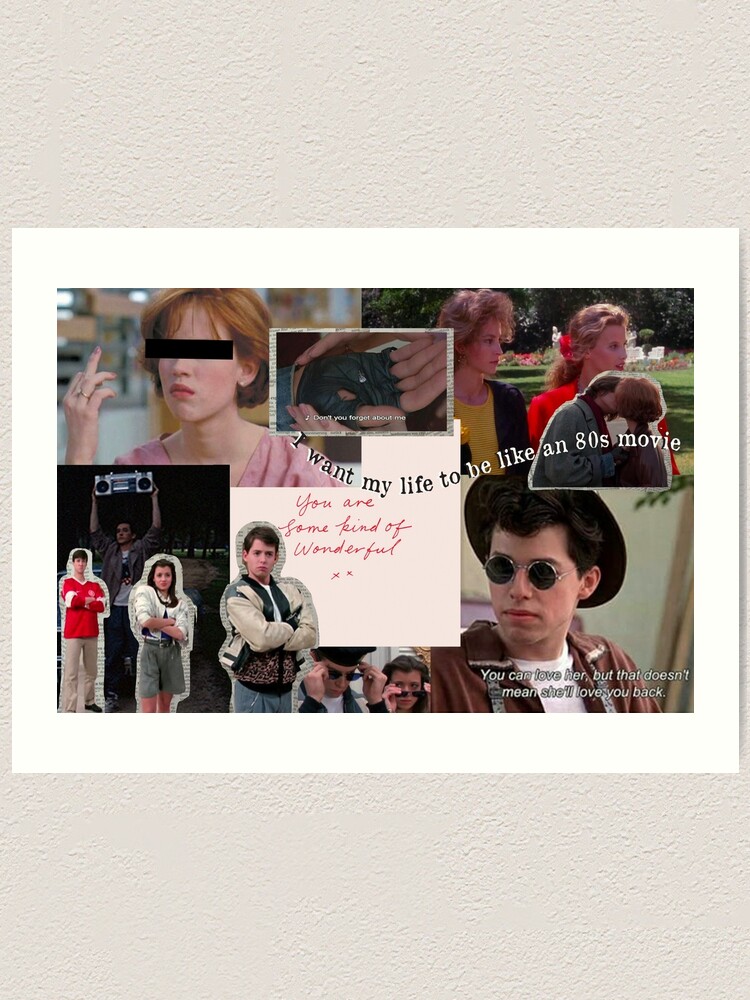The image is a vibrant collage of iconic scenes from 80s movies, with an emphasis on films featuring Molly Ringwald and other beloved teen film stars of the era. Central to the collage is a redacted image of Molly Ringwald from "The Breakfast Club," where her eyes are obscured by a black bar as she gives the finger. Another notable still from the same movie showcases Molly Ringwald kissing the notorious bad boy of the story. 

In the middle of the collage, a distinctive image captures a hand wearing fingerless gloves, delicately holding an earring, also from "The Breakfast Club." Another memorable scene features John Cusack from "Say Anything," immortalized as he stands with a boombox hoisted above his head. 

Interspersed among these scenes are images from "Ferris Bueller's Day Off," including the three main characters—Ferris, Sloane, and Cameron—cut out from the art gallery scene. Additional images from the movie capture more iconic moments of Matthew Broderick as Ferris. 

The collage includes a charming still from "Pretty in Pink," highlighting another memorable character. Text overlays add a wistful narrative to the collage with phrases like "I want my life to be like an 80s movie," "You are some kind of wonderful," and "You can love her but that doesn't mean she'll love you back." The color palette of the image is rich, featuring black, white, gray, red, pink, orange, green, blue, silver, and peach, enhancing the nostalgic and retro feel of the montage. The characters' clothing further emphasizes the vintage, old-school vibe characteristic of 80s fashion.